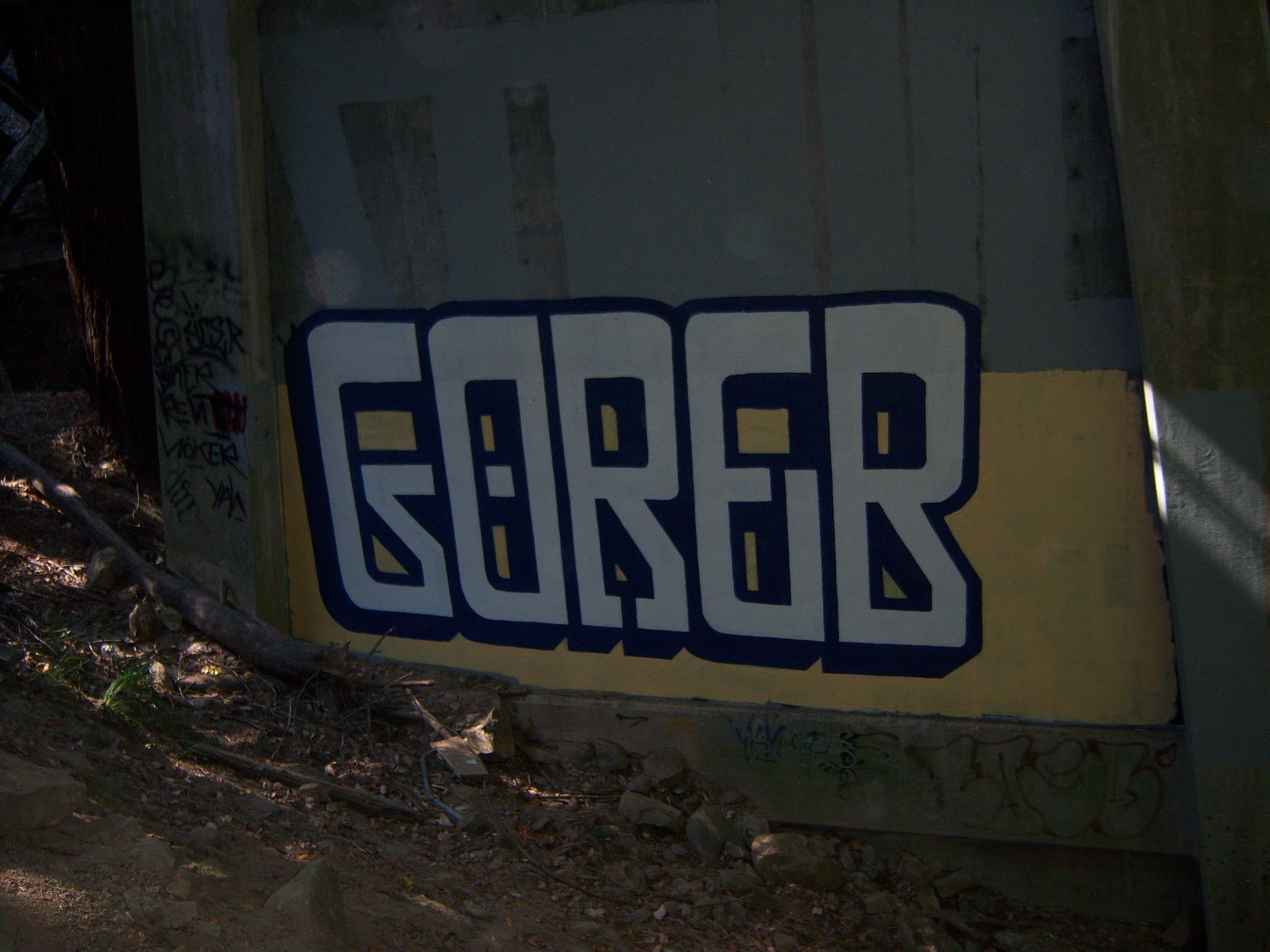The photograph depicts a dark, likely nighttime scene featuring a dirty, gray concrete wall that seems to be part of an outdoor structure, possibly under a bridge. Centered on the wall, there is graffiti in white block letters spelling "G-O-R-E-R," neatly outlined in blue paint against a yellow background. The surrounding area on the wall is marred by additional, less intricate black graffiti and general grime. Below and in front of the wall, the ground slopes and is scattered with tan-colored dirt, rocks, sticks, and strewn leaves, giving the impression of a neglected space under a bridge.